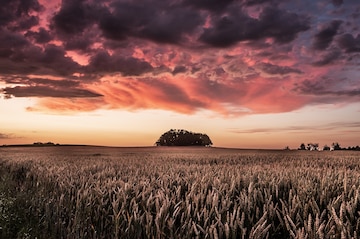The image depicts a stunning rural landscape during golden hour or sunset, likely in the Midwestern United States. The foreground is dominated by a vast field, possibly wheat or a similar crop, with tall stalks and silky tops. The central focus is a large, full green tree or perhaps a dense cluster of trees standing prominently in the distance. Surrounding this central tree, the horizon reveals a faint and distant white farm or house, complemented by tiny, scattered green trees and potential structures, like barns, towards the right edge of the photo. The sky above is a captivating gradient of colors. At the top, dark purple clouds give way to various shades of pink, creating a banded effect with some orange outlines. A light strip of sunlight underlines the clouds, transitioning into a peach-hued skyline that meets the vibrant, though grayed, grass of the field. The entire scene is subtly shaded by a dark or gray filter, enhancing the serene and tranquil ambiance of the sunset.